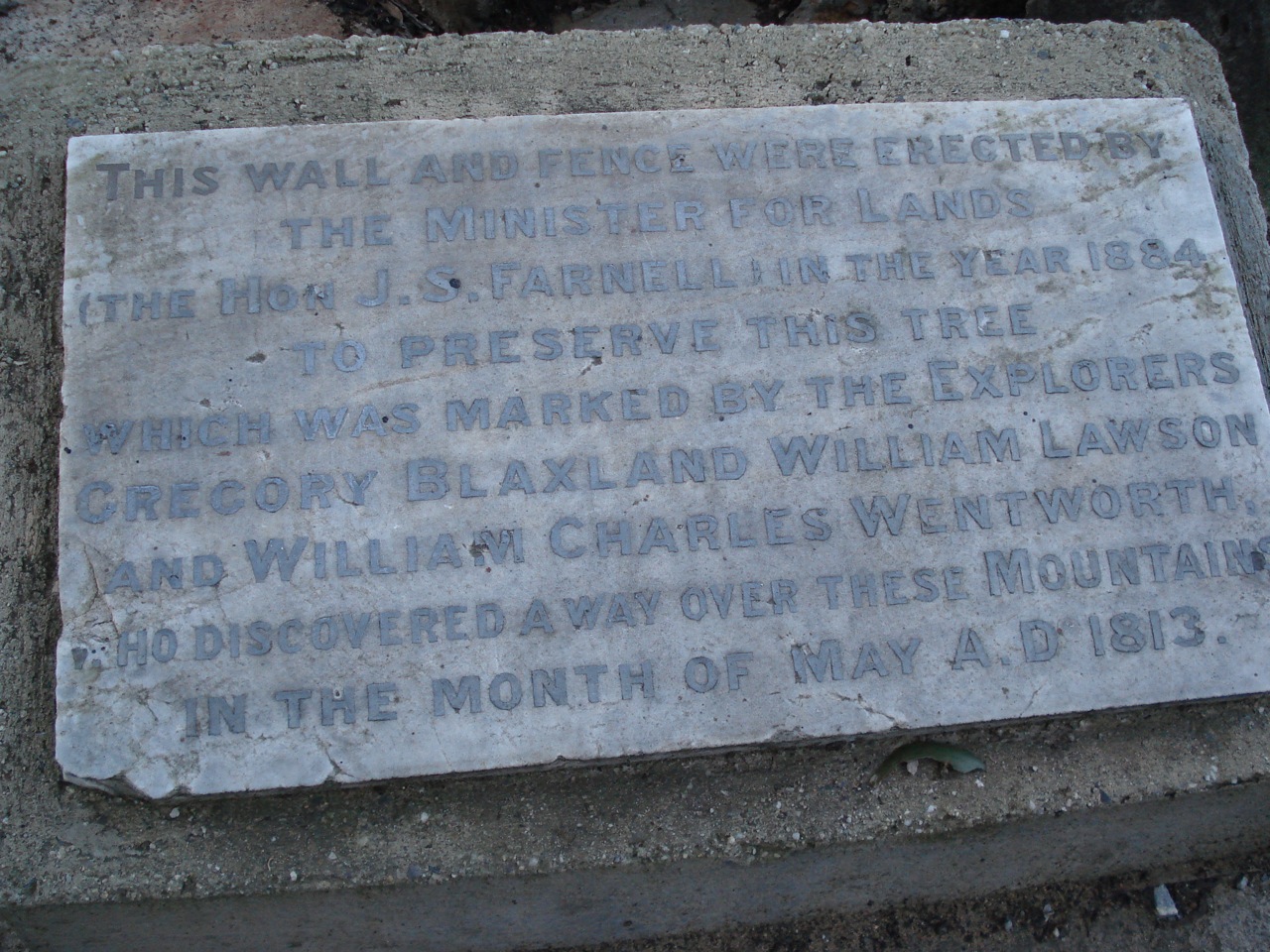The image features a weathered, off-white concrete plaque affixed to a grey stone that is part of an unseen larger wall. The plaque, which appears to be slightly angled upwards and situated on the ground amongst some dirt, bears light blue or silver lettering. This text is noticeably faded and partially worn away, making it difficult to read. The inscription on the plaque states: "This wall and fence were erected by the Minister for Lands, the Honourable J.S. Farnell, in the year 1884 to preserve this tree, which was marked by the explorers Gregory Blaxland, William Lawson, and William Charles Wentworth, who discovered a way over these mountains in May, A.D. 1813." Though the stone backdrop is largely hidden by the plaque, its grey, concrete-like texture is evident. The entire setup gives a sense of historical significance but is marred by dirt, cracks, and the wear of time.